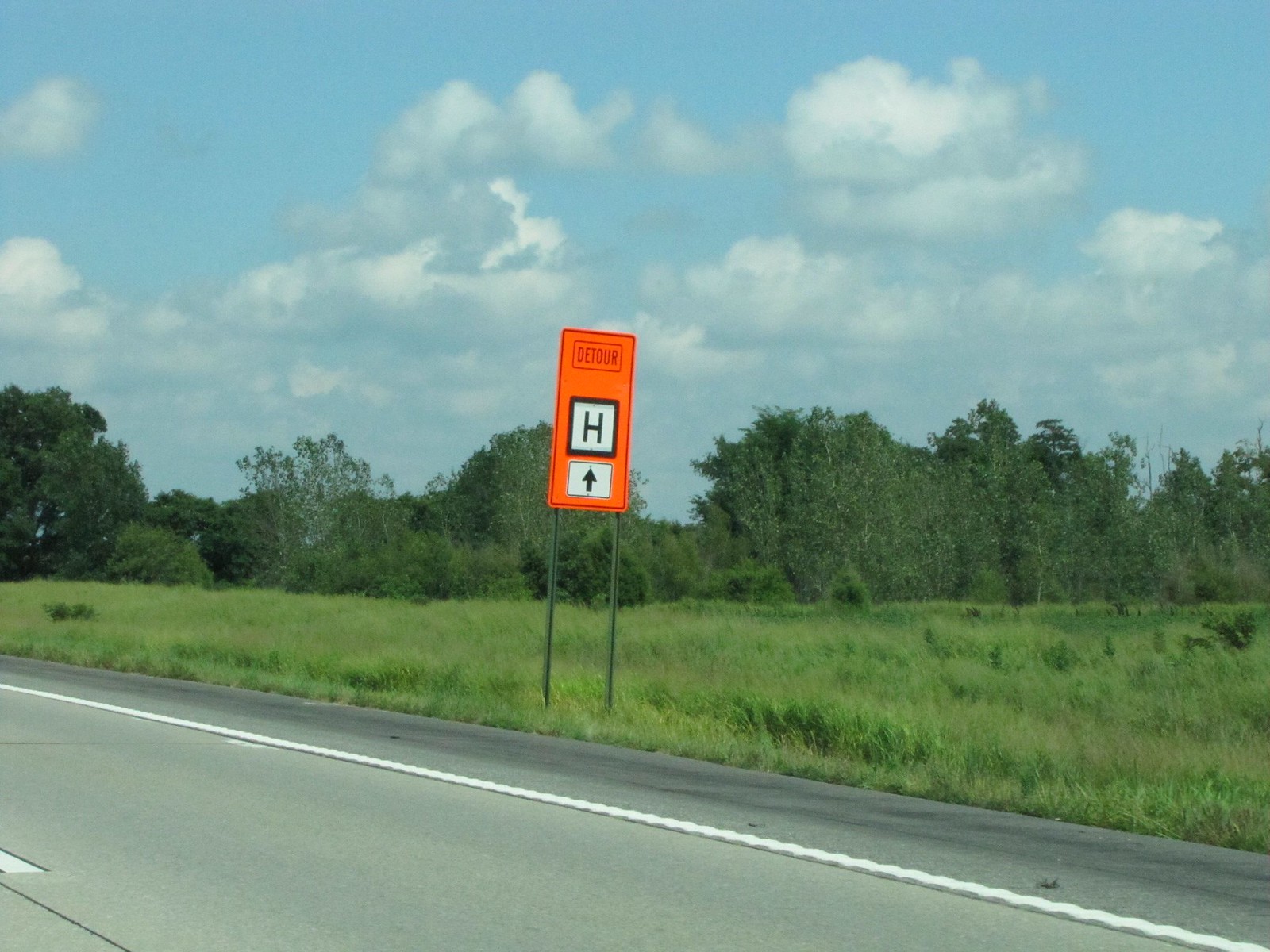The image captures a scenic highway scene dominated by a prominent, orange detour sign. The tall, skinny rectangular sign features the word "detour" at the top in black lettering encased within a rectangular box. Beneath it, a white square holds a capital "H" in black, mounted against a backdrop of black trim, likely indicating Highway H. Below the "H" box, a black arrow points straight ahead. The sign is supported by two metal poles rooted in a grassy meadow beside a two-lane highway. This highway, constructed of typical blacktop, features a dotted center line and a white line at the shoulder, flanked by a corrugated edge meant to alert drivers when they veer off course. The surrounding landscape includes a field of tall grass and weeds leading up to a line of trees that extends across the image. The sky above is a blend of light blue with large, fluffy gray and white clouds, creating a picturesque yet functional roadside view.